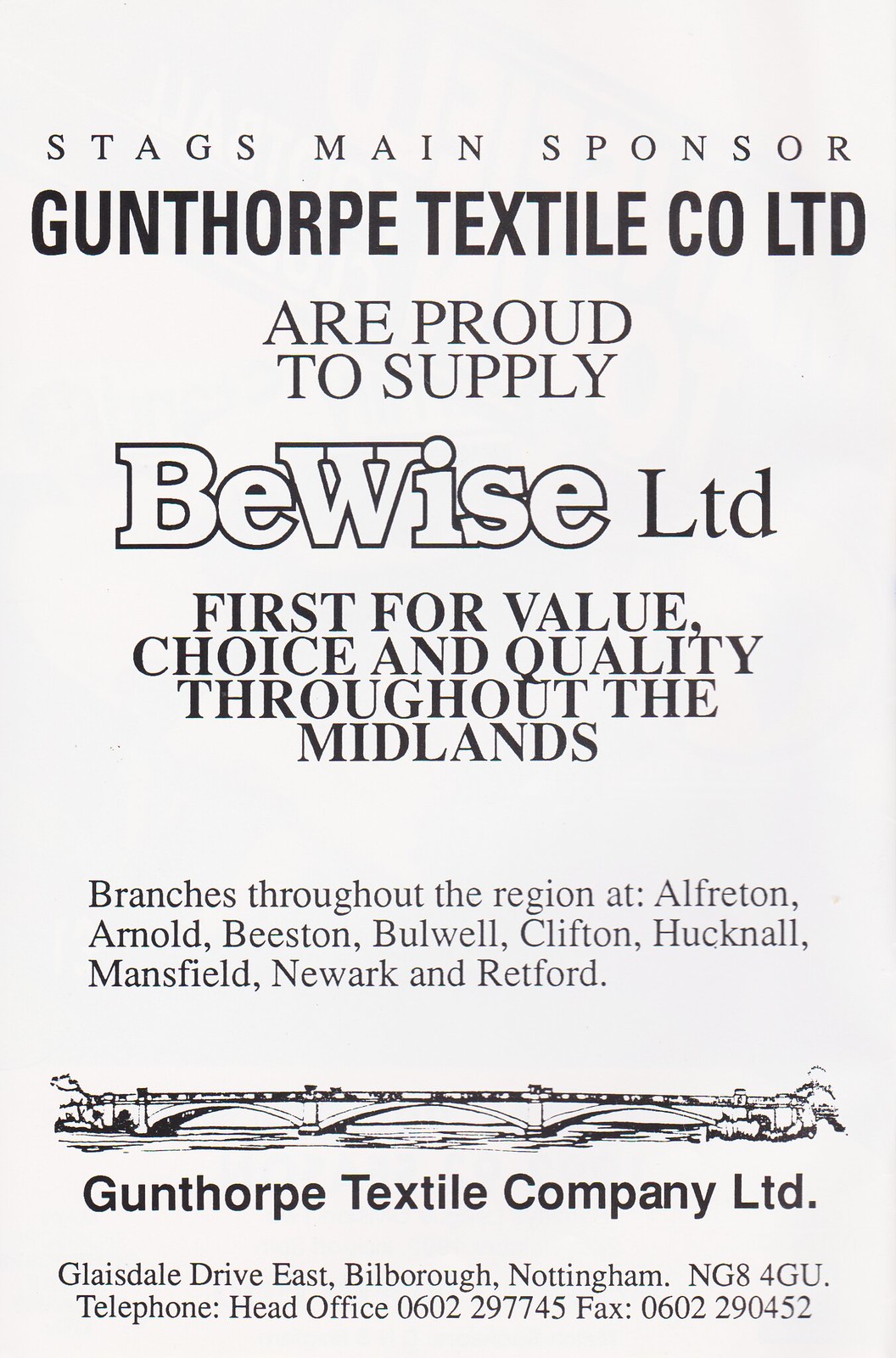This image is a black-and-white advertisement flyer for Stagg's main sponsor, Gunthorpe Textile Company Limited, displayed in bold black text on an off-white or pale blue background. At the very top of the flyer, "Staggs Main Sponsor" is prominently featured. Below it, the text reads: "Gunthorpe Textile Company Limited are proud to supply Be Wise Limited, first for value, choice, and quality throughout the Midlands." In the latter half of the flyer, it lists the locations of Gunthorpe Textile Company's branches, which are in Alfredton, Arnold, Beeston, Bulwell, Clifton, Hucknall, Mansfield, Newark, and Retford. Near the bottom, there is a thin, elongated graphic of a bridge spanning from left to right. Below this graphic, the text reaffirms the company's name, Gunthorpe Textile Company Limited, followed by the address and contact details: Glazedale Drive East, Bilborough, Nottingham, NG8 4GU, Telephone: Head Office 0602-297745, Fax: 0602-290452.